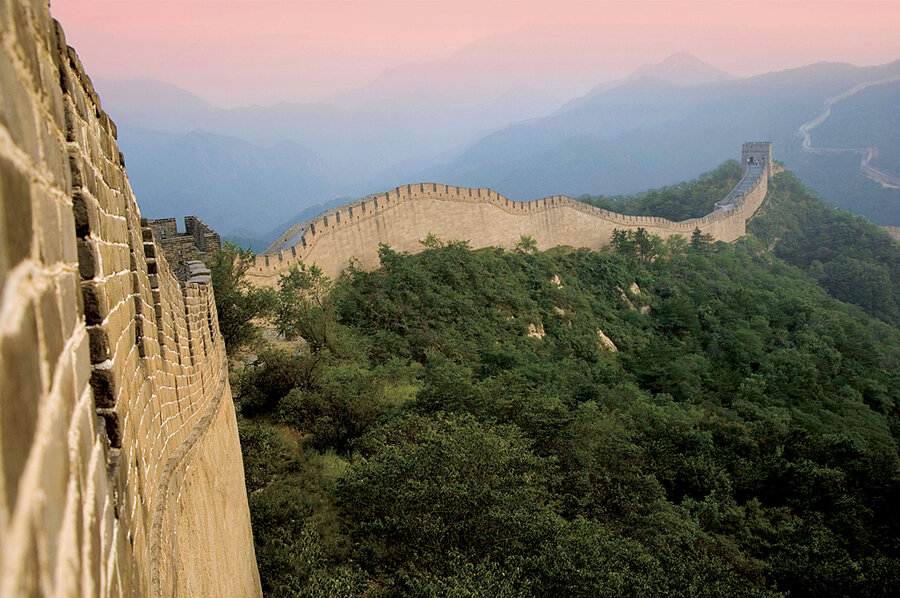This image captures a breathtaking view of the Great Wall of China as it stretches across a lush, green landscape dotted with dense trees and bushes. The ancient Wall, built of rustic brownish-beige bricks, stands prominently against the vibrant greenery that envelops it. The Wall's immense length is highlighted as it winds its way into the distance, showcasing its grandiose and historic architecture. Above the scene, the sky is an extraordinary gradient, fading from a foggy pink at the top to deeper shades of blue, hinting at the onset of dusk or dawn. The distant horizon is lined with majestic mountains, their peaks faintly visible through the atmospheric haze, further accentuating the Wall's imposing presence in this enchanting natural scene.